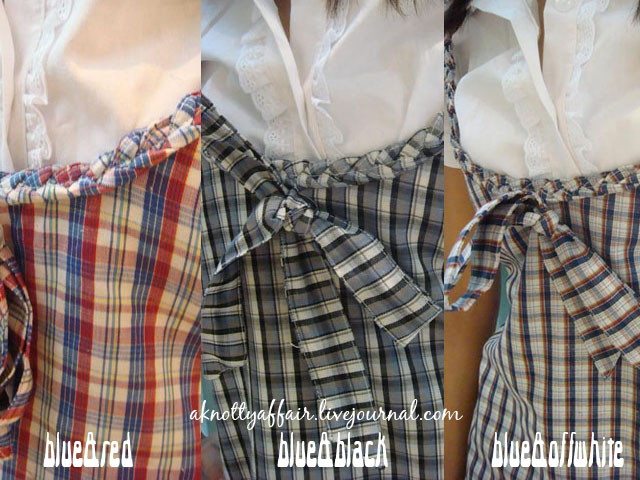This image showcases three separate, split-view photos of a white, ruffled shirt paired with different plaid skirts. Each skirt features a distinct color pattern and design details. The left skirt displays a blue and red plaid pattern with a ruffled top, while the middle skirt showcases a blue and black plaid design, similarly ruffled and accented with a bow. The right skirt features a more complex pattern with blue, off-white, and a brown stripe, again with a ruffled top and a bow. The outfits are worn by a person, as strands of hair and part of an arm are visible, suggesting it's not a mannequin. The backdrop, partially obscured by the clothing, appears to be a brown wall. Notably, the image contains a label, "a naughtyaffair.livejournal.com," indicating a branding or promotional element.